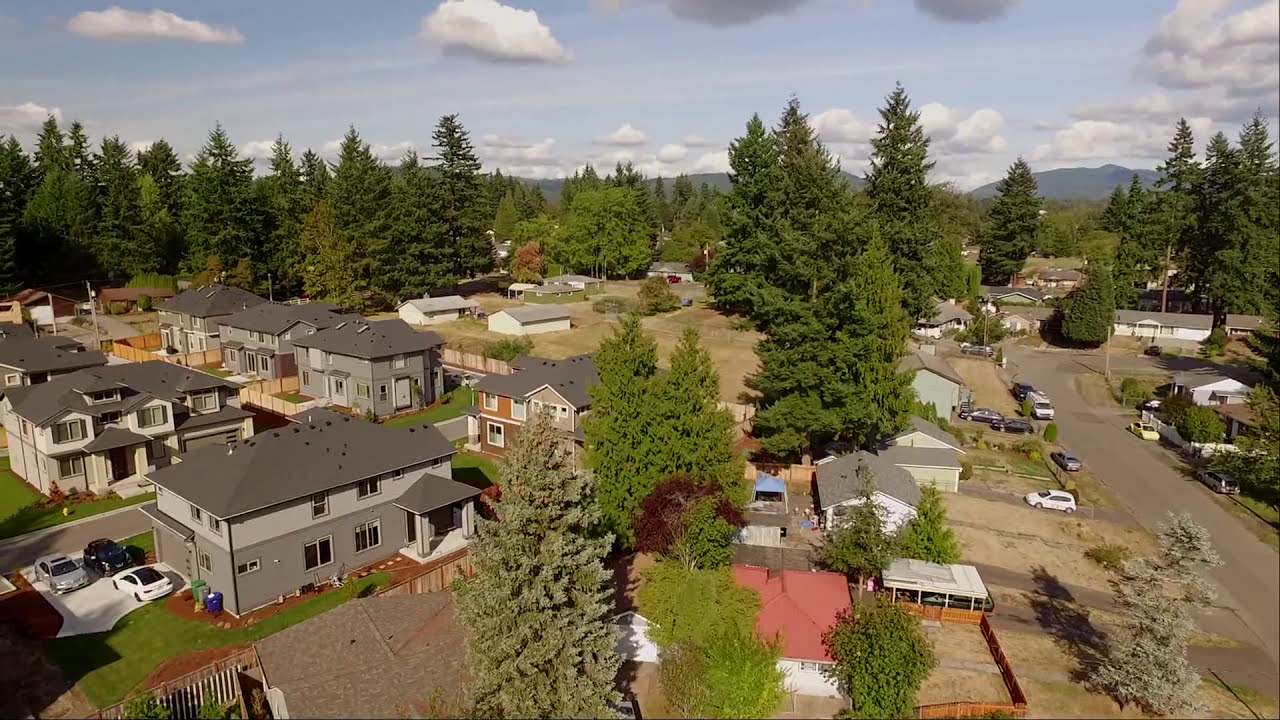This vibrant daylight aerial photograph captures a picturesque neighborhood, likely taken by a drone from a height equivalent to six or seven stories. The image features a blend of large evergreen pine trees and residential structures set against a clear blue sky with scattered fluffy white clouds. On the left side, there is a cluster of visually similar two-story houses painted in light or drab gray tones, with neatly maintained green lawns. The house closest to the camera has three cars - a gray, a black, and a white one - parked in its driveway. In contrast, the right side of the image reveals a collection of smaller, single-story homes, and outbuildings lined along a winding street. These houses also have driveways with several parked cars. Separating these areas are numerous pine trees that add a lush green canopy to the scene. In the center, an open field or a slight elevation change disrupts the road’s visibility, creating a natural focal point. Stretching into the distance, forested hills or mountains provide a stunning backdrop, completing this detailed and serene depiction of a well-established and possibly affluent neighborhood.